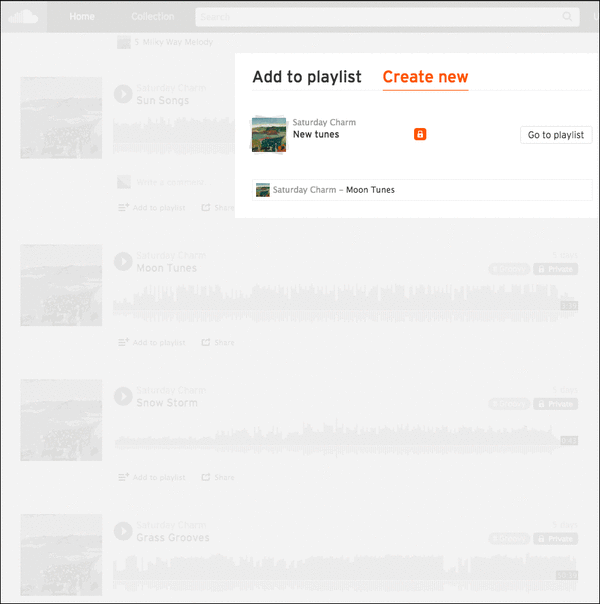This detailed caption describes elements visible in a cropped screenshot of the SoundCloud desktop web page, providing insights into the user interface:

"The screenshot depicts a portion of the SoundCloud desktop web page with a semi-transparent dark gray overlay. Centered towards the top of the screen is a prominent white box, with the phrase 'Add to Playlist' displayed in large black letters at the top-left corner. Adjacent to this, 'Create New' is written on the top-right, highlighted in orange font with an accompanying horizontal orange underline, indicating it is selected.

Inside the white box, towards the bottom left, there is a thumbnail of an album cover. To the top-right of this cover, the text 'Saturday Charm' appears in small gray letters. Below this text, 'New Tunes' is stated in bold black letters. Centrally located within this white box is a small orange square featuring a white padlock icon.

On the far right inside the white box, there is a small gray-outlined button labeled 'Go to Playlist' in gray letters. Additionally, at the bottom left, another gray outlined rectangle encompasses a secondary album cover thumbnail in the bottom left corner. Above this album cover, 'Sunday Charm' appears again in small gray letters, and 'Moon Tunes' in bold black letters.

In the background, partially obscured yet discernible, is the faint outline of the SoundCloud logo situated in the top left corner."